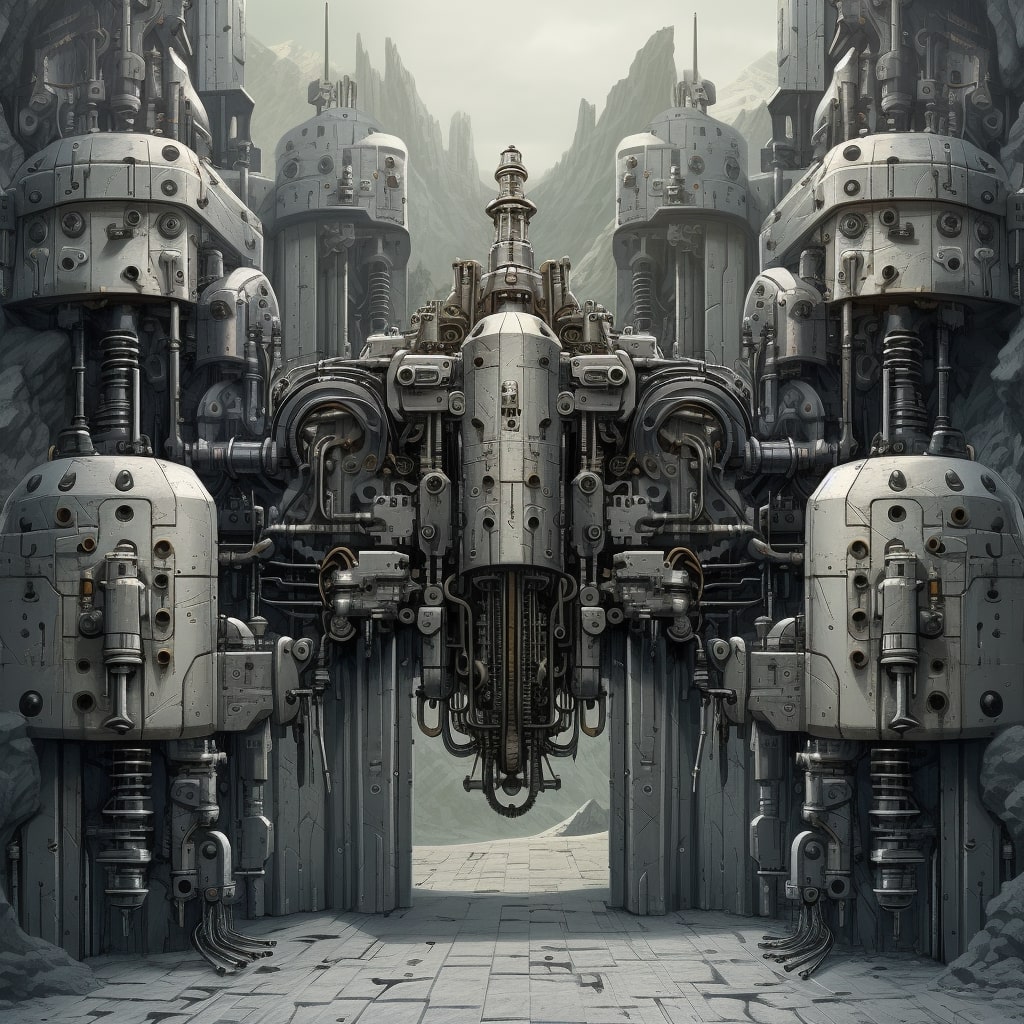The image depicts a large, square, steampunk-styled mechanical gate set against a backdrop of gray, clouded sky and distant mountain peaks. Dominating the foreground are cylindrical metal tanks, with notable ones on the left and right appearing identical, raised above the ground and featuring coil mechanisms at their bases. Centered within the composition is a prominent, narrower cylindrical structure adorned with metal projections that connect it to the nearby tanks. This central piece creates an archway under which a pathway formed from irregular, rectangular, and square gray stones winds through, hinting at the possibility of passage to the other side. The entire scene is enveloped in shades of gray and brown, contributing to its distinctly industrial and mechanical aesthetic.